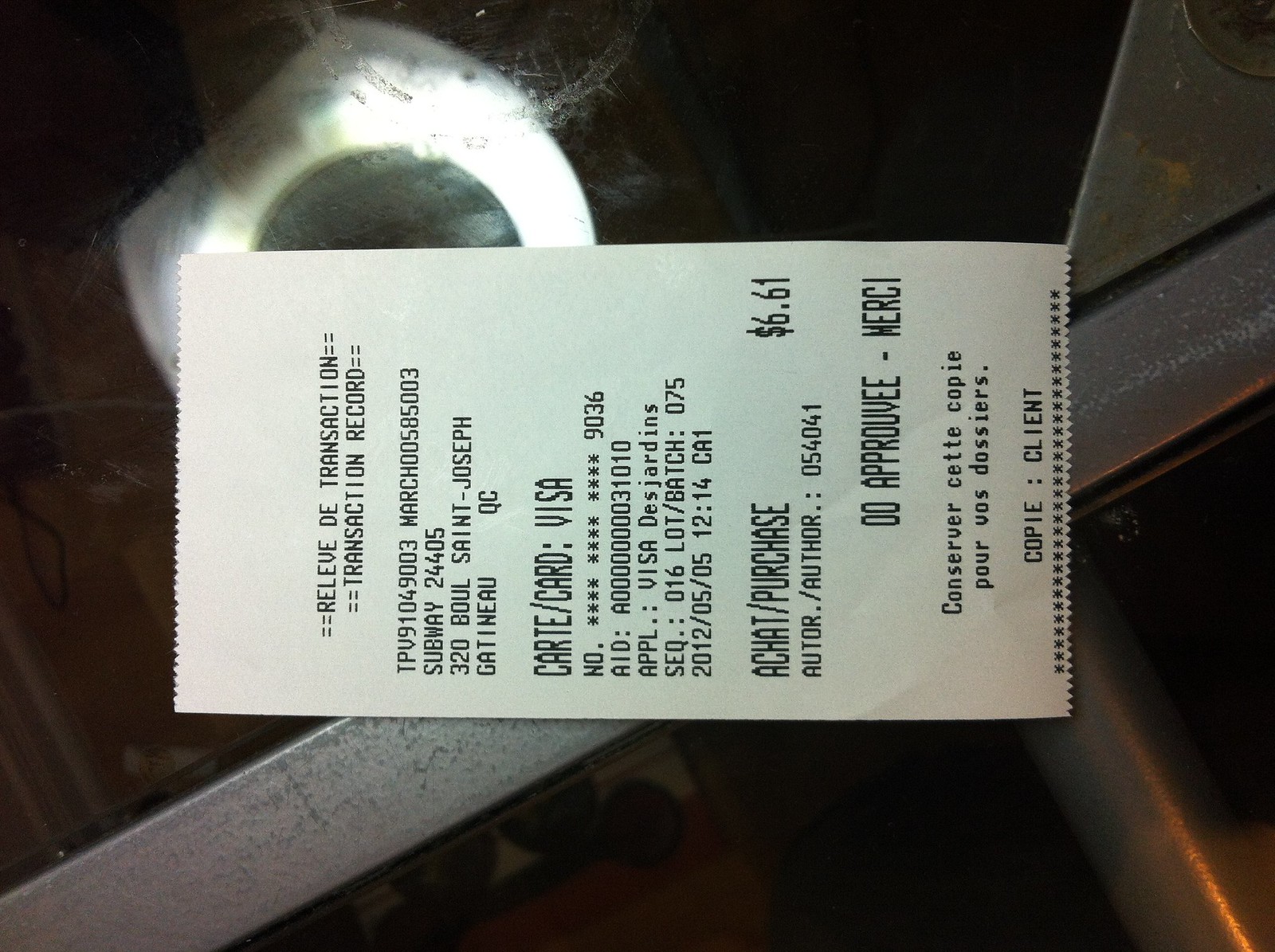A photograph captures a crinkled, bright white receipt with crisp black printing, labeled "Relieved to Transaction, Transaction Record." The receipt, issued by Subway location 24-2405, shows a total of $6.61. It sits slightly askew atop a clear, glass table with worn, stained metal edges, giving an industrial vibe. The glass surface is marred by dust and smudges, obscuring the details of objects underneath. Part of the receipt hangs over the table's edge, revealing a dark, indistinct background that might be a carpeted floor. Additionally, a blurry white cylindrical object lies beneath the glass, contributing to the scene's gritty texture.